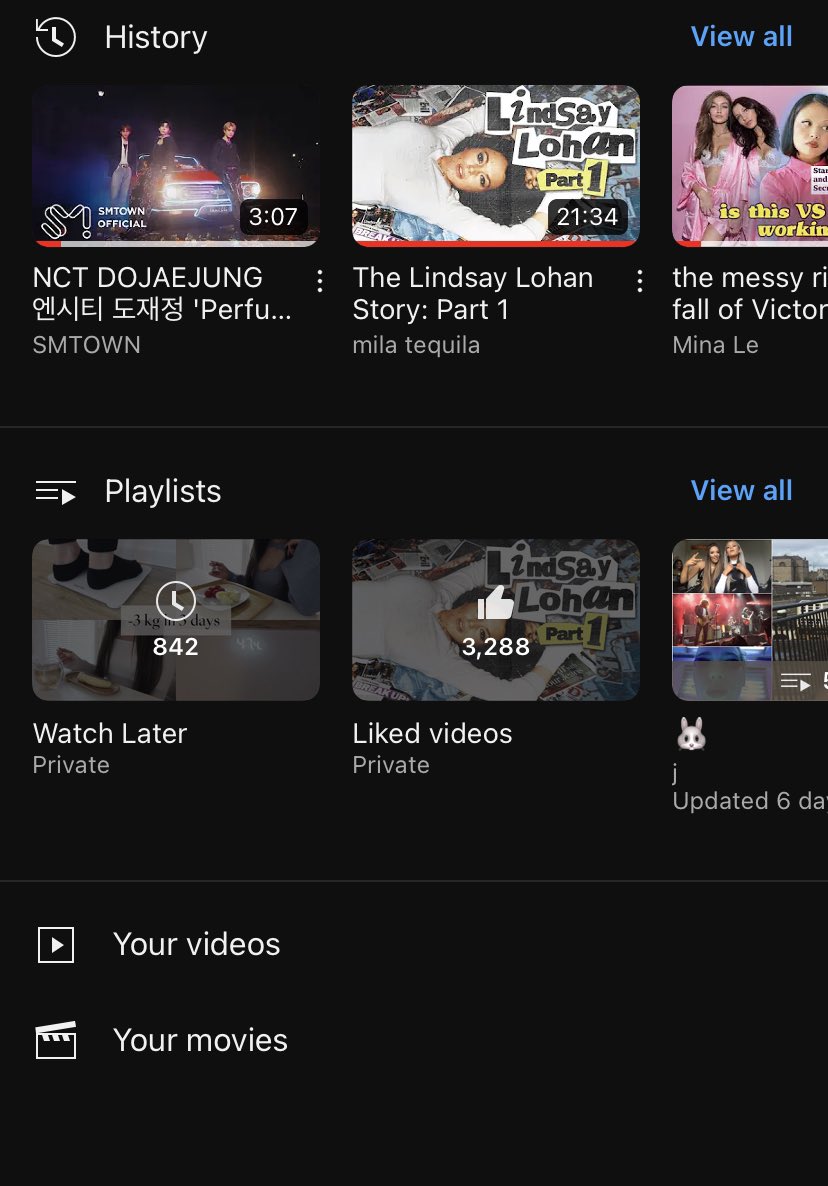Here's a cleaned-up and detailed caption based on the provided description:

---

A partial screenshot, likely captured from a tablet, of a video-sharing website akin to YouTube or Rumble. The screen displays a section titled "History" at the top, showcasing thumbnails for three videos: one 3 minutes and 7 seconds long, another 21 minutes and 34 seconds, and a partially visible third one. Below this, there's a section with "Playlists" featuring two categories: "Watch Later" with 842 videos and "Liked Videos" with 3,288 videos. The screen's layout includes navigation options such as "Your Videos" and "Your Movies." The interface is sleek, characterized by a black background with white text, giving it a modern and user-friendly appearance.

---

This caption provides a comprehensive and clear description of the screenshot contents.